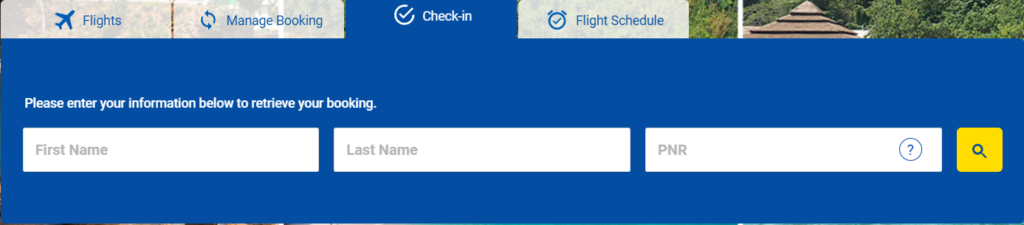In this image, we see a detailed flight booking page. The interface prominently features options such as "Flights," "Categories of Flights," "Manage Booking," "Check-In," and "Flight Schedule." Beneath these categories, there is a user input section prompting travelers to enter their booking information. The required fields include "First Name," "Last Name," and "PNR (Passenger Name Record)." Adjacent to these fields is a bright yellow search button adorned with a magnifying glass icon for easy access, as well as a help icon marked by a question mark. The overall color scheme of the page employs a combination of blue, white, and yellow, lending a visually appealing and clear layout.